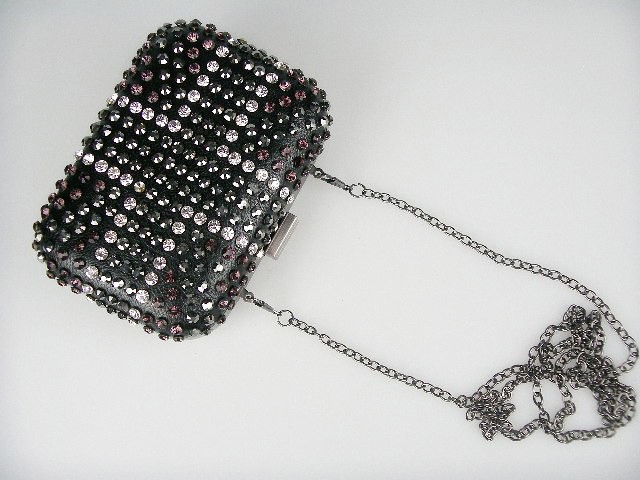The image showcases an elegant, evening purse set against a pristine white background. The purse, rectangular in shape and designed for fancy occasions, features a long silver chain strap that lies crumpled to the right of the purse. The purse itself is a striking black, adorned with a cross made from white gemstones that outline the cross, with green gemstones filling in the cross and red gemstones adorning the outer edges. Additionally, the purse includes intricate beadwork with black, silver, and pinkish purple beads, adding to its luxurious appearance. A small silver buckle is also visible, enhancing its sophisticated and opulent design. The photograph, taken from above, captures the detailed craftsmanship and refined elegance of this stunning accessory.